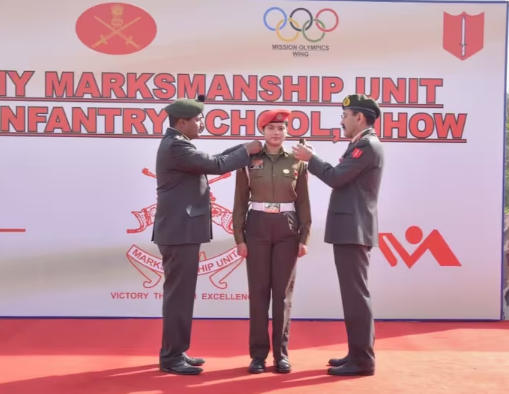In this detailed image, we see a proud moment captured during an award ceremony, likely taking place in India despite the English text. Central to the photograph is a female soldier standing at attention, adorned in a brown military uniform with a white belt and a red beret. She is being honored by two senior officers, both dressed in dark greenish-gray military attire and matching caps. Together, they are placing badges onto her shoulders, recognizing her achievements.

The backdrop features a white wall with prominent red text reading "Marksmanship Unit, Infantry School." Various emblems and logos are also visible, including the Olympic rings at the top, signifying the association with "Mission Olympics Wing". Additional text such as "Victory Excellence" supports the theme of high achievement in marksmanship. The ground they stand on is an orangish-red carpet, which adds to the ceremonial atmosphere of the scene.